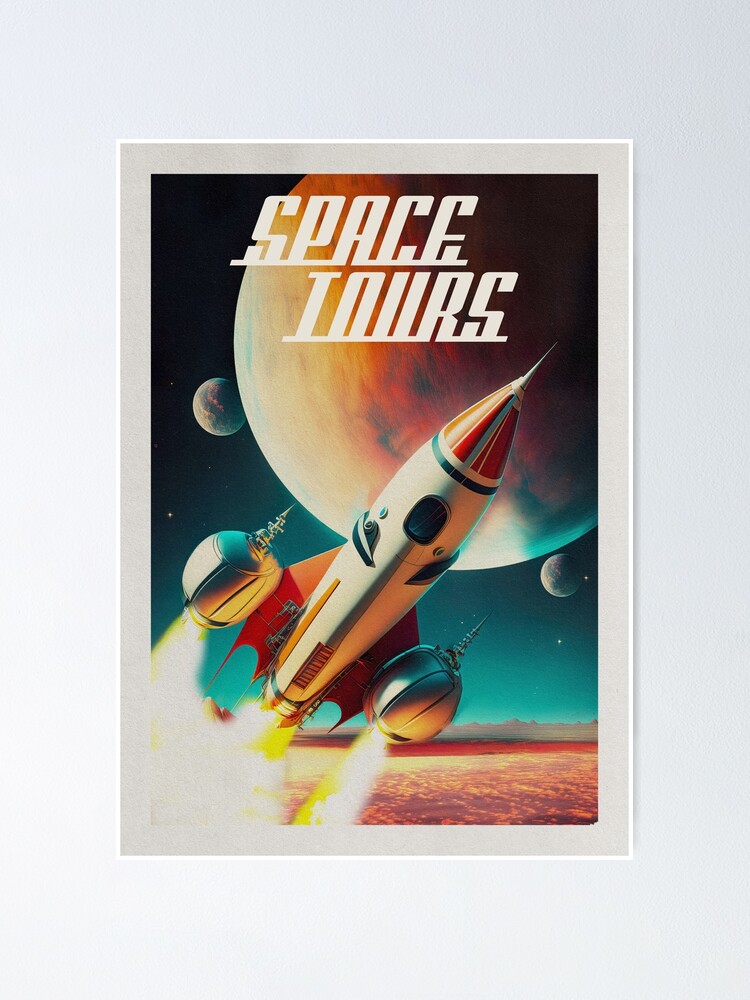This is a detailed illustration of a "Space Tours" poster, presented in a white frame against a pale grey wall. The print prominently showcases a stylized rocket ship blasting off from the bottom-left corner with vibrant trails of fire. The rocket, characterized by its sharp, pencil-like shape with red, blue, yellow, and green elements, ascends towards a dark, space-themed background, transitioning from black and deep blue at the top to teal and brownish-red near the bottom.

At the top of the poster, the words "Space Tours" are boldly displayed in a bright, white, space-themed font. Behind the rocket, there's a large, visually stunning planet with predominant reddish-orange and yellow hues, partially off-frame towards the top right. Accompanying this major planet are two smaller planets with bluish tones, positioned respectively to the left and underneath the larger planet, creating a sense of depth and cosmic scenery.

Stars are speckled across the dark expanse, enhancing the celestial ambiance of the artwork. The poster's overall aesthetic is reminiscent of a vintage travel advertisement, with a modern sci-fi twist, making it perfect for a youthful, indie-styled space or anyone with a love for space exploration and artistic décor.